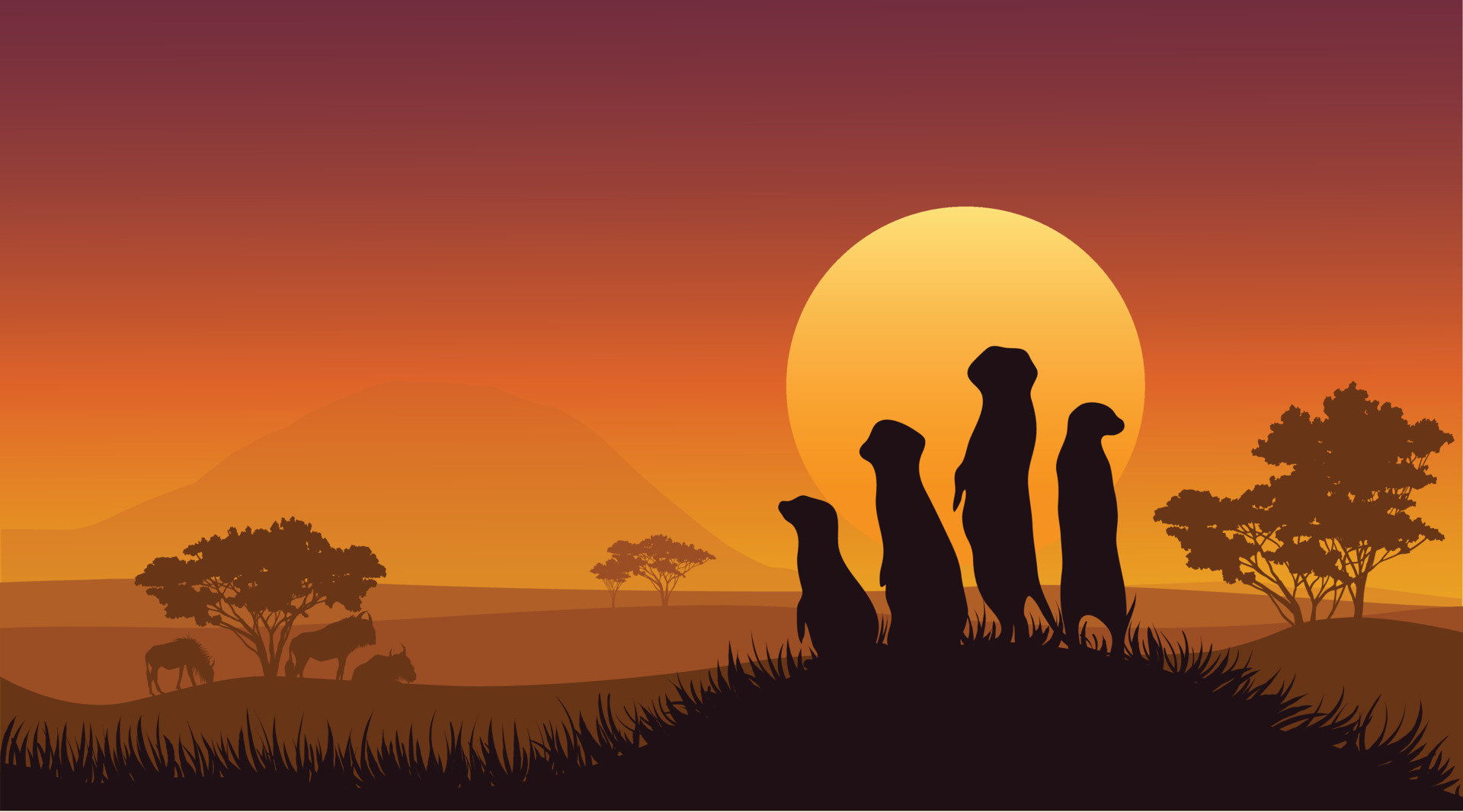This horizontal, computer-generated image presents a captivating silhouette scene of four prairie dogs standing upright on their hind legs atop a grassy hill, directly facing a large, brilliant yellow sun set against a stunning rust-orange sky. The detailed silhouettes of the prairie dogs, complete with short paws and tufted grass beneath them, add to the charm of the scene. In the background, there is a faint silhouette of a mountain range on the left and four trees dotting the landscape—one to the far left with three grazing horses beneath it, one in the center, and one to the right, which has leaves and sits on a small hill. Farther back, under one of these trees, three buffalo can be seen, enhancing the depth and beauty of this serene prairie sunset.